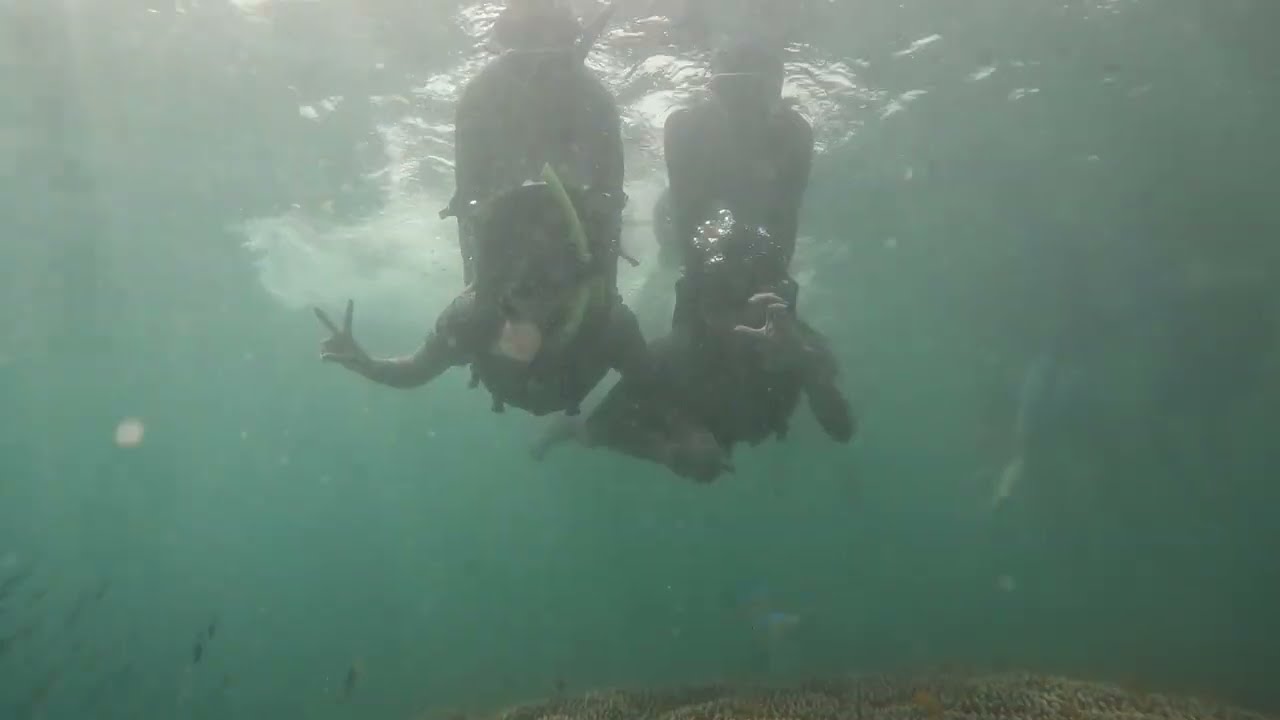In the murky, greenish-yellow water, a group of four scuba divers is captured mid-dive. The visibility is low, but shafts of light pierce through from above, creating a dappled effect on the scene. Central to the image are two divers descending toward the ocean floor—one on the left is making a victory sign with his fingers, while the diver on the right appears to be forming a C-shaped motion with his hand. Above these two, partially obscured, are two more divers, their forms faint against the hazy background. Bubbles rise around them, likely from their tanks, adding to the underwater ambiance. Below, coral or gravel and possibly some sea creatures, contribute to the textured ocean floor. The divers' gear glints subtly in the ambient light, adding to the intrigue of this underwater tableau.